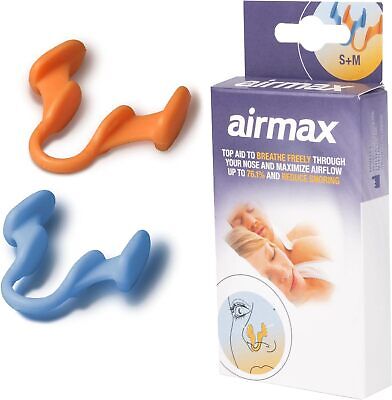The image features a product designed to aid breathing during sleep by inserting into the nostrils to maximize airflow and reduce snoring. The right side prominently displays the packaging of the product, labeled "Air Max." The upper part of the box is light purple, transitioning to white at the bottom. It includes a large text that reads "Air Max" at the top and "Top aid to breathe freely through your nose and maximize airflow up to 76.1% and reduce snoring" below. 

On the front of the box, there's a photograph of a Caucasian couple, a man and a woman, both sound asleep on white pillows. The man appears slightly unshaven, and the woman has dirty blonde straight hair. Below this photo, there is a black pen-and-ink line illustration depicting the nasal device, which consists of two yellow inserts placed into a nose to demonstrate its application.

To the left of the packaging, the image shows two plastic nasal devices; one is larger and orange, while the other is smaller and light blue. These devices feature two inserts with rounded tips and wedged fins to ensure they fit snugly inside the nostrils, and they both possess a rounded rectangular base for easier insertion and removal. The top of the box also indicates the sizes available, marked as "S + M."